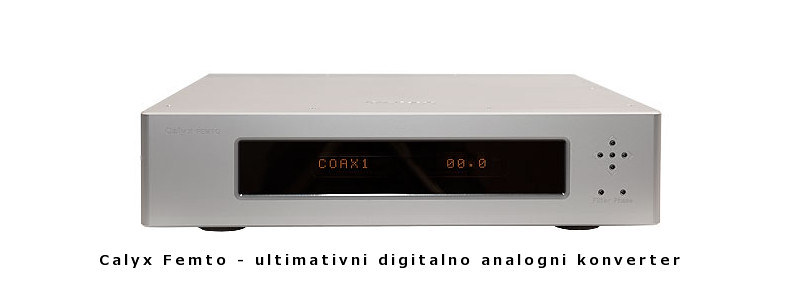This image showcases a professional advertisement of a metallic silver digital converter box, resembling the shape and size of a VCR or a CD/DVD player. This sleek device features a central black screen with "Coax 1" on the left, followed by "00.0" in orange digital text. Positioned to the right of the screen are five multi-functional buttons arranged in a diamond shape, with additional buttons beneath them. The device rests on small black protrusions at its base, giving it a sturdy appearance. Marked prominently along the bottom in black text are the words "Calyx Femto-Ultimativni Digitalno Analogni Konverter," indicating its multifunctional capabilities. The text is partially in a different language, emphasizing the product's universal appeal and advanced technology.